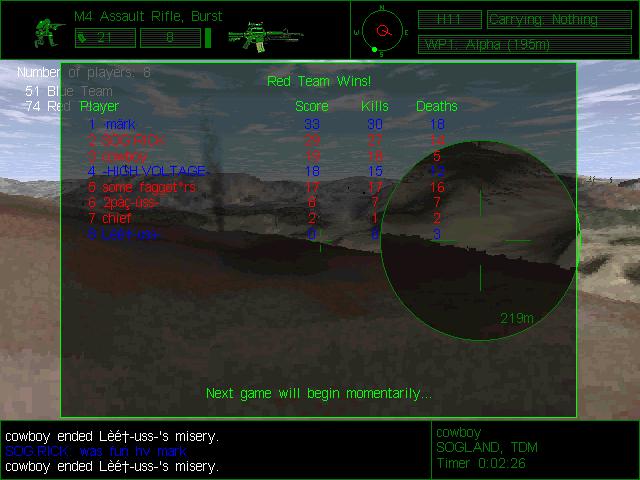The image is a captured screenshot from a first-person shooter video game, displaying the end-of-match scoreboard. Dominating the center of the screen is a translucent green-bordered square with the text, "Red Team wins," at the top. Below this, the columns headed "Player," "Score," "Kills," and "Deaths" present the results, with player names and their respective stats listed in blue and red text, although the details appear somewhat distorted.

At the bottom of the screen, the message "Next game will begin momentarily" signals an imminent new round. The bottom right corner of the screen shows the green text, "Cowboy, SOGLan, TDM, timer 0.02.26." The bottom left corner features a chat box in black, including the text "Cowboy ended Elite USS' misery" in white.

The top left corner displays "M4 Assault Rifle, Burst," alongside an image of a crouched figure holding a gun. Meanwhile, the top right corner indicates, "H11, Carrying, Nothing, WP1 Alpha (195 meters)." The background visible through the green-bordered square suggests a desert terrain with mountainous landscapes, plumes of black smoke, and a sky filled with elongated white clouds.